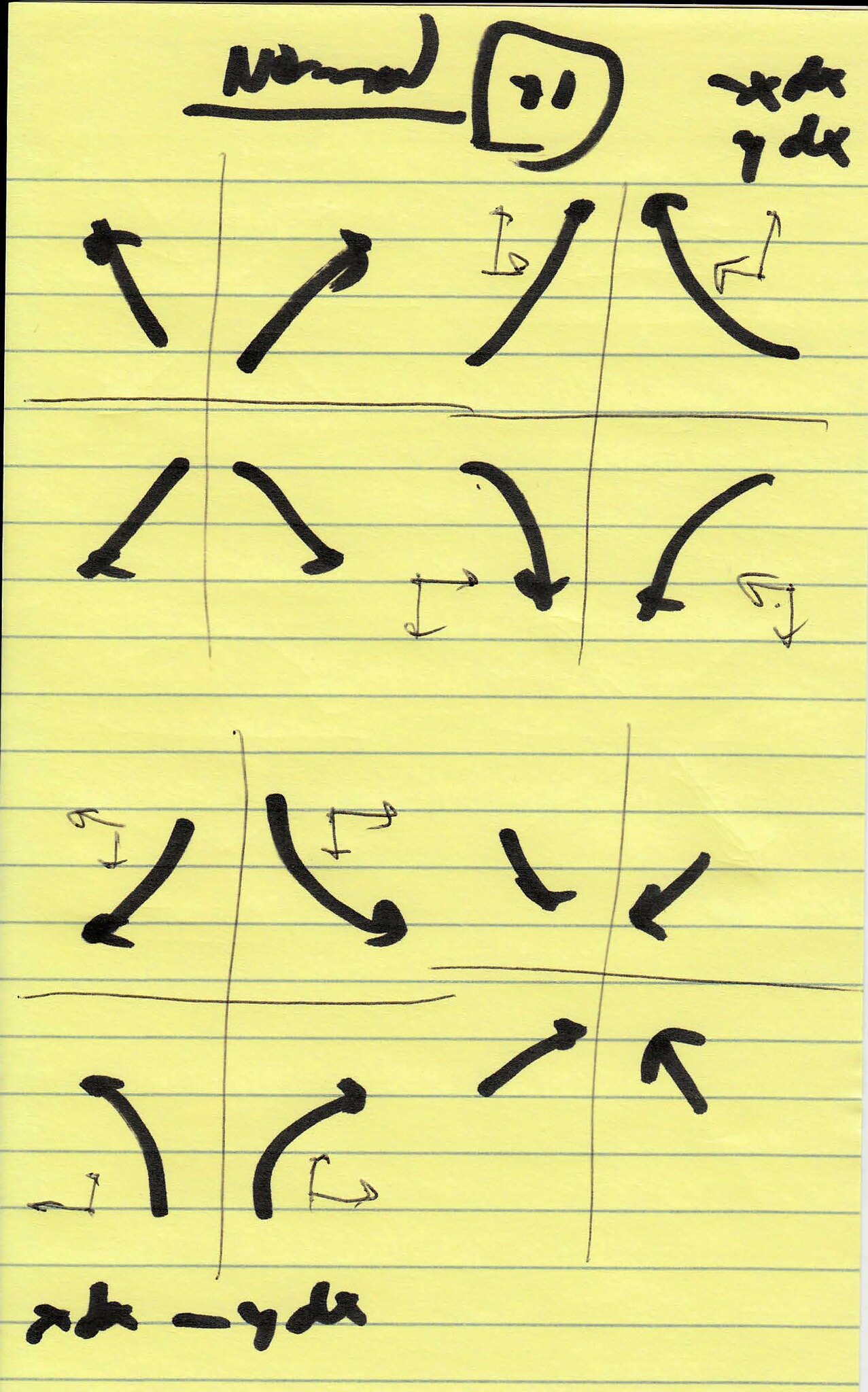This color photograph features a vertically oriented yellow lined legal pad. At the top of the pad, there is a section of illegible scribbled writing. Additionally, the top of the pad contains a hastily drawn square with two thick, black vertical lines inside it. The bottom of the square is slightly open. In the top left corner of the page, several arrows are drawn diagonally pointing in various directions: left, right, down-left, and down-right. Adjacent to these arrows are other arrows that curve inward, and further down, there are arrows that curve outward, with this pattern mirrored at the bottom of the pad in the opposite direction. Scattered across the page, there are scribbled lines resembling clock hands. Both black marker and black ballpoint pen have been used for the writing and illustrations. The image is devoid of people, animals, plants, flowers, trees, and buildings, focusing solely on the chaotic and somewhat enigmatic diagram on the legal pad.